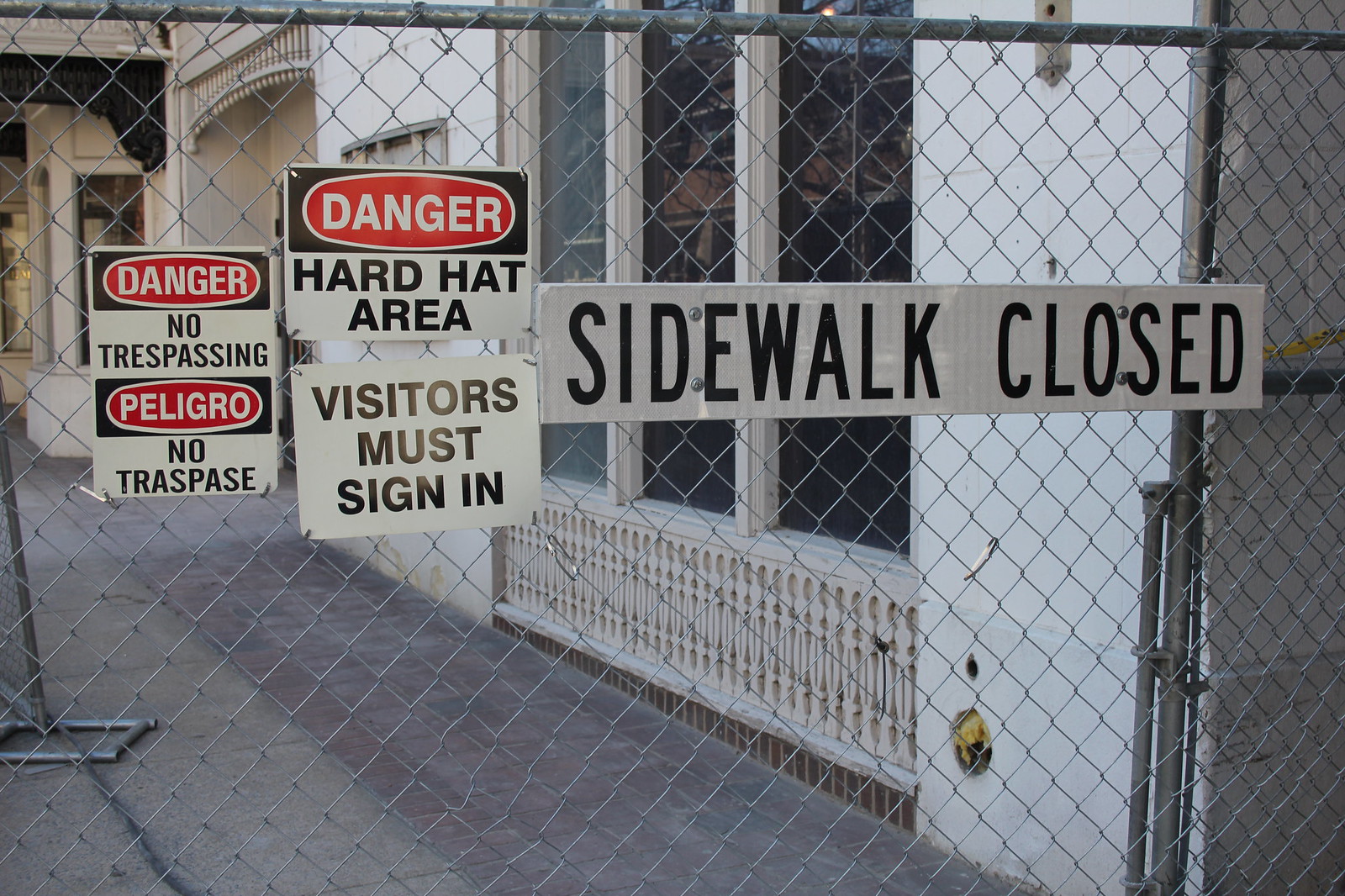The image features a prominent metal mesh gate in the forefront, adorned with multiple warning signs. Centrally placed on the gate, these signs read: "Danger, No Trespassing," repeated in Spanish as "Peligro, No Traspase," "Danger, Hard Hat Area, Visitors Must Sign In," and a large rectangular sign stating "Sidewalk Closed." The gate and signs are the focal point of the image, with the colors red, white, black, gray, yellow, and a touch of silver standing out. In the background, through the gate, a white building with three large windows is partially visible, accompanied by a walkway. The setting appears to be outdoors, likely during midday, and seems to be within a construction zone, given the hard hat area warning. Additionally, there's another piece of fencing visible further in the background on the sidewalk.